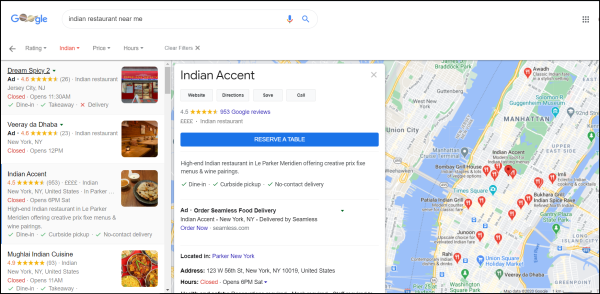The image depicts a Google search results page for "Indian restaurant near me." The main Google logo at the top is adorned with playful designs; the two O's are illustrated as planets in blue, yellow, and red colors. Below the search bar, which prominently features a blue and red microphone icon, and a blue magnifying glass icon for search, appears a list of Indian restaurants.

At the top of the list, there's a filter for rating with a dropdown arrow beside it. Highlighted in red text is "Indian" followed by the word "Dream" with a rating of 4.6 stars. A note indicates it is currently closed and will open at 11:30 AM. The next entry, "Vooray Di Dabda" in New York, New York, holds a 4.5-star rating, is closed, but will reopen at 12:00 PM. Following that, "Indian Accent," also rated 4.5 stars, is closed and set to open at 6:00 PM on Saturday. Lastly, "Mughlai Indian Cuisine" boasts a 4.9-star rating and is expected to open at 11:00 AM.

The user appears to have selected "Indian Accent" for a table reservation, as indicated by the highlighted blue bar showing options like dine-in and curbside pickup.